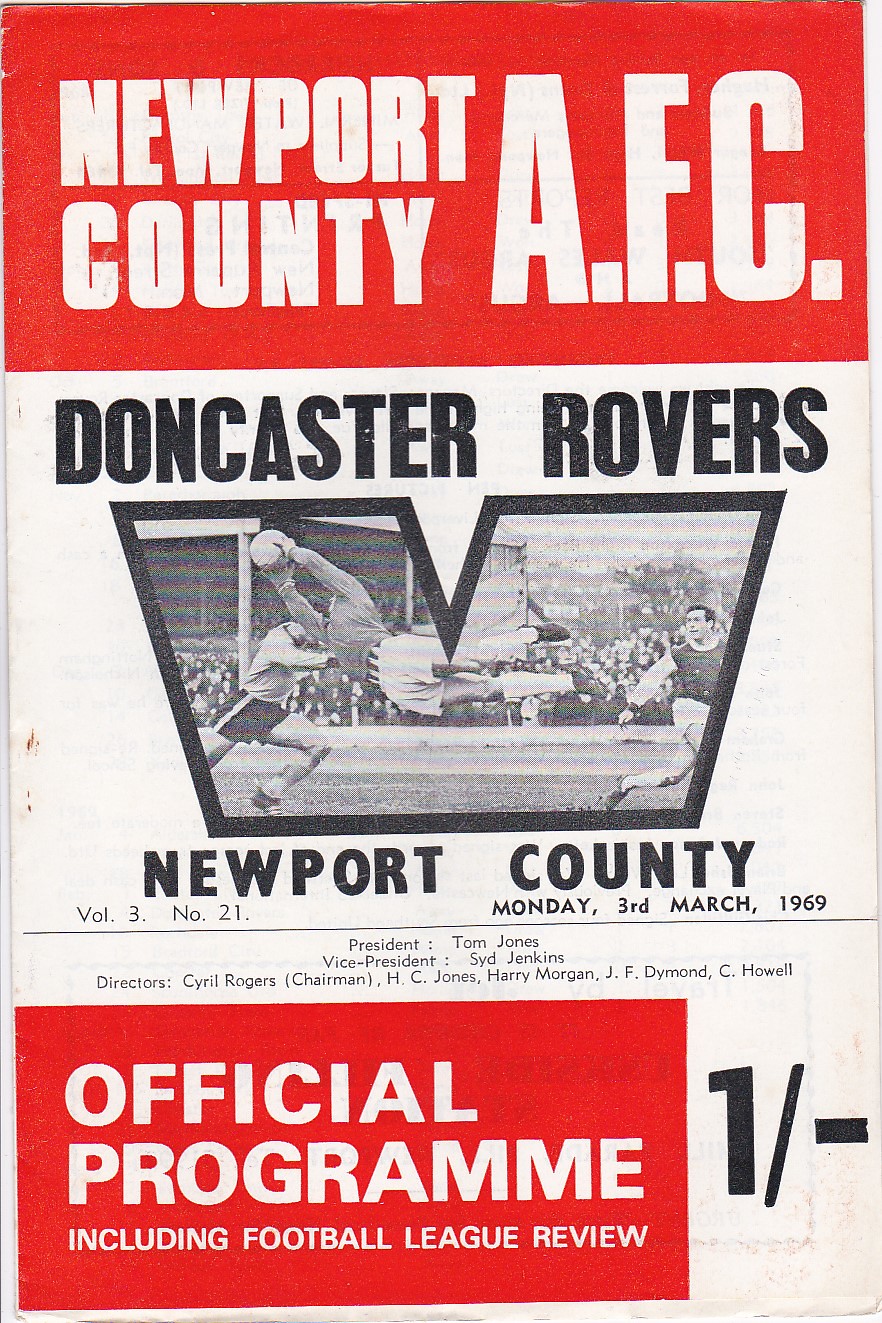The cover of the official program for the Newport County AFC vs. Doncaster Rovers soccer match presents a visually striking design in red, white, and black. At the top, a red background hosts "Newport County AFC" in bold, white capital letters. Below it, a white section displays "Doncaster Rovers" in large, black capital letters, followed by a prominent letter 'V'. Inside this 'V' is a black-and-white photograph depicting an intense soccer moment: a goalie in a dark uniform is leaping to the left with outstretched arms to catch a white soccer ball, while two other players, one in a light uniform and the other in a darker one, sprint across the field. The crowd can be seen in the background. Below the 'V', "Newport County" is also printed in bold, black capital letters. The bottom section features a red background with white text reading "Official Program, including Football League Review." In the lower corner, it provides additional details such as volume number 3, issue number 21, and the date, Monday 3rd March 1969. The program lists names of officials including President Tom Jones, Vice President Sid Jenkins, and others, with a small "1/-" in the bottom right corner, denoting its price.